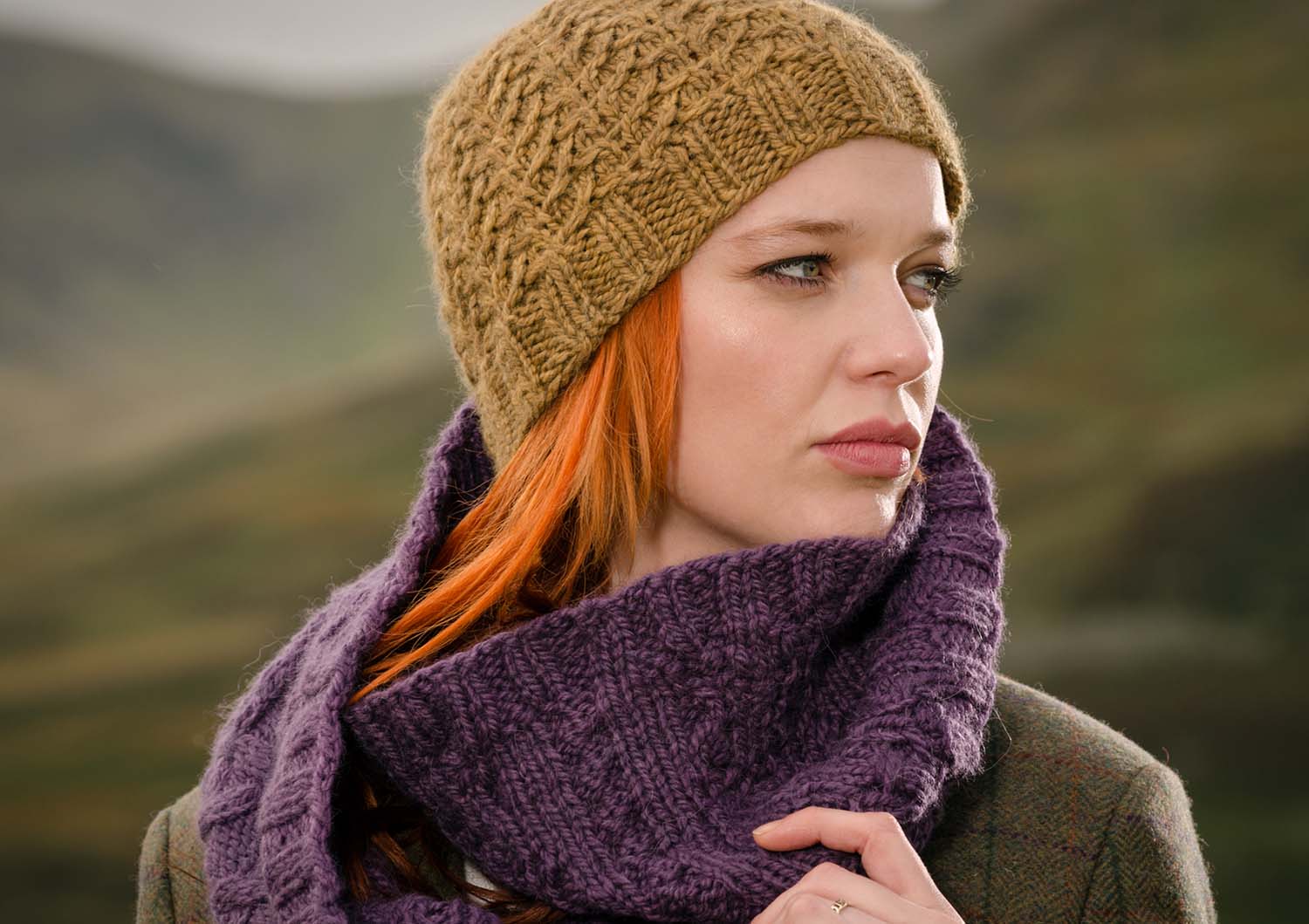The image captures a close-up, professional photograph of a young woman with striking, bright reddish-orange hair, peeking out from under a light brown, hand-knit toboggan. She has white skin and is positioned centrally in the horizontal rectangular frame against a background that blends various shades of brown, possibly depicting a blurred mountainside. Her head is sharply turned to the left, gazing off into the distance, revealing her well-applied makeup with pink lipstick and eye makeup. She is adorned with a deep purple, hand-knit scarf that wraps around her neck and drapes down her right side, and she appears to be dressed in the top portion of a suit jacket or wool blazer. Her hand is partially visible, gently holding the edge of the scarf, and she wears a gold ring on her finger. The photo has a product shot quality, possibly highlighting the knitted accessories she wears.